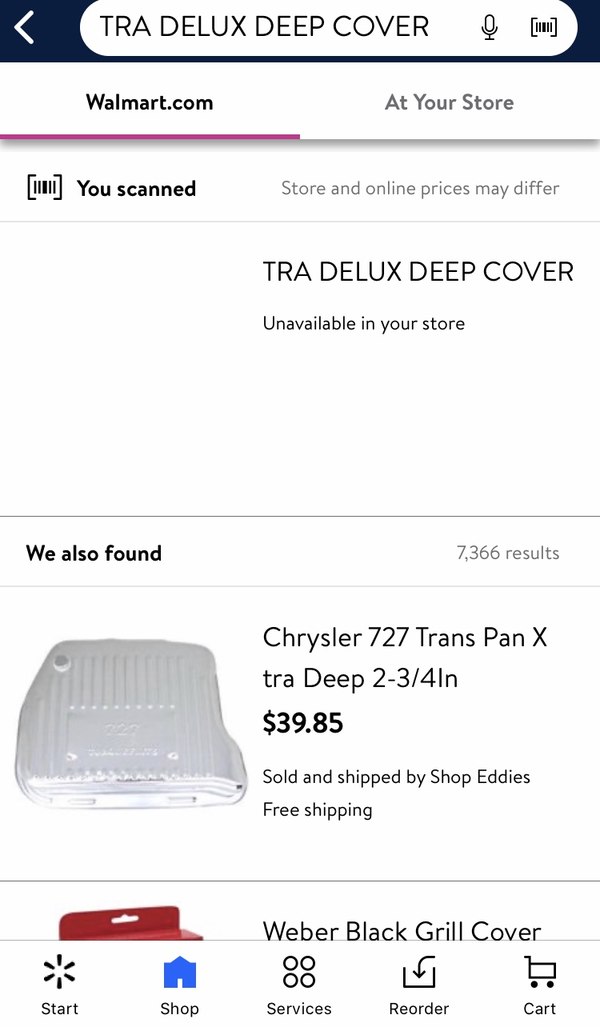The webpage depicted in the image displays a search query for "TRA DELUX DEEP COVER" at the top, with the search term spelled out in capital letters. Beneath the search bar are two navigational tabs: "Walmart," which is bolded with a red underline to signify it as the active tab, and "At Your Store," which is grayed out, indicating it is inactive. Just below these tabs, the phrase "You Scanned" is shown next to a barcode icon, accompanied by a note stating, "Store and Online Prices May Differ."

Further down, the product title "Troth Deluxe Deep Cover" is displayed prominently, followed by a notification that the item is "Unavailable in Your Store." Following a small amount of white space and a horizontal divider, the section labeled "We Also Found" appears, alongside the number "7,366 results," indicating alternative related items.

Highlighted among the search results is a gray-colored image of an automotive part, labeled "Chrysler 727 Transpan Extra Deep 2-3 1/4." The item is priced at $39.85, and additional details mention it is "Sold and Shipped by ShopEddy's" with "Free Shipping."

At the bottom of the screen are icons representing various services available on the webpage: starting from the left, a Walmart icon labeled "Start," a blue house icon labeled "Shop," followed by an icon for "Services" denoted by four dots arranged in a square, an icon labeled "Reorder" with a box and arrow symbol, and finally, a cart icon with the word "Cart" beneath it.